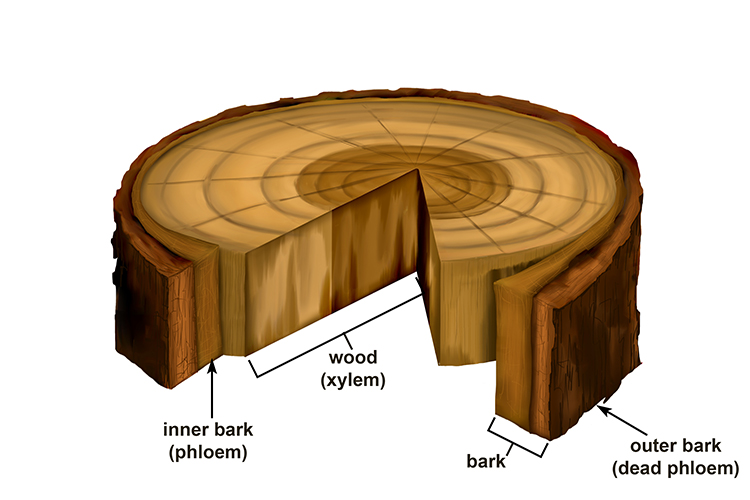The diagram illustrates a cross-section of a tree trunk, showcasing a detailed examination of tree rings and layers of bark. The section appears to be about six inches in diameter, with a visible wedge-shaped segment excised to expose the internal structure.

On the right side, an arrow points to the "Outer Bark," annotated with the term "Dead Phloem" (P-H-L-O-E-M) in parentheses. Adjacent to this, another label indicates the "Bark," distinguishing two distinct layers: an outer reddish-brown layer and an inner, darker layer.

On the left side of the diagram, an arrow indicates the "Inner Bark," labeled as "Phloem" in parentheses. Below this inner bark is the region labeled "Wood," which is further identified as "Xylem" (Z-Y-L-E-M) in parentheses.

The xylem features two different colorations: an outer section consisting of four lighter brown rings and an inner section of three rings that closely match the hue of the inner bark. Notably, the pie-shaped missing segment and the slightly peeled-away bark on the right side highlight the distinction between the tree's layers.

This comprehensive illustration serves to provide an insightful look into the intricate layers and growth patterns of a tree.